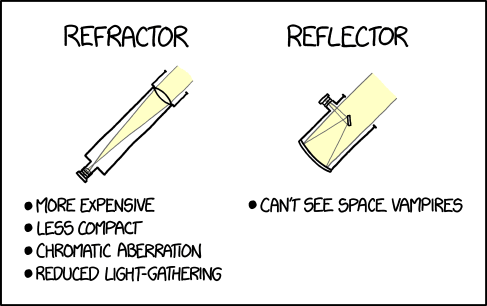The image depicts a comparative diagram of two types of telescopes: a refractor and a reflector. On the left side, labeled "Refractor", an illustration shows a light beam passing through a lens. Accompanying bullet points indicate the key characteristics: "More expensive," "Less compact," "Chromatic aberration," and "Reduced light gathering." The text highlights these disadvantages twice for emphasis.

On the right side, labeled "Reflector," a graphic illustrates light being directed into a reflective device, which then bounces the light. The only listed attribute for this type on the diagram humorously states, "Can't see space vampires." 

Both sections of the image feature white text on a background with black borders, using visual markers like bullet points to organize the presented information.